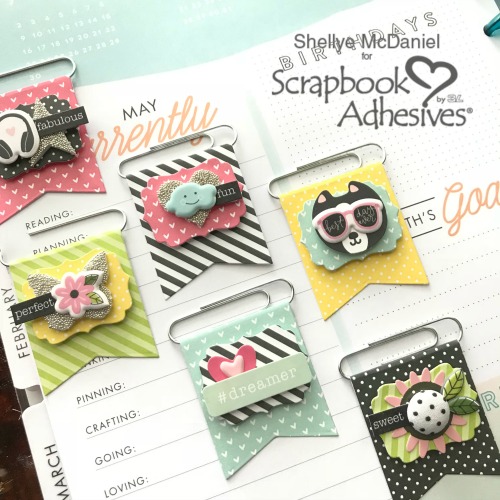This is a detailed advertisement mock-up for scrapbook adhesives designed by Shelly McDaniel. The image, computer-generated, showcases a colorful and vibrant set of upgraded stickers, resembling small banners, each attached to paperclips and placed on a calendar or address book. The focal point includes various playful elements: a dog with sunglasses, flowers, hearts, clouds, and earphones. Each sticker features a specific design and message: a ball with a flower saying "sweet," a heart with "dreamer," clouds with a heart saying "fun," another flower with "perfect," and earphones with "fabulous." The colors are predominantly pastel shades of greens, pinks, yellows, and whites. Each banner-shaped sticker has its unique pattern and colors, like pink with light pink hearts, black and white stripes, dark green and light green stripes, yellow with white polka dots, blue with white hearts, and black with white polka dots. The top right corner of the image features black lettering saying "Shelly McDaniel for Scrapbook Adhesives" with a heart accentuating the 'i' in adhesives, emphasizing the creative and personal touch of the product design.